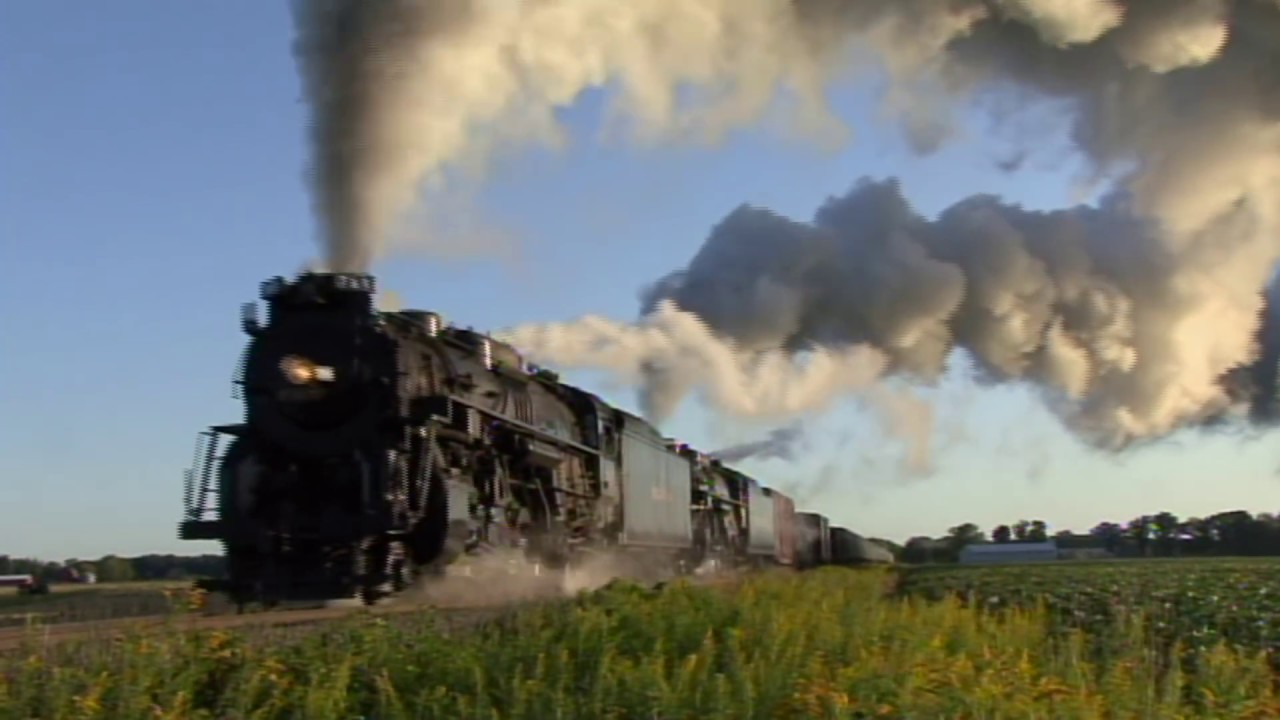This photo appears to be a dramatic still from a movie or television show, capturing a black steam locomotive from an older era, similar to what you might find in a Wild West setting, in full motion on the tracks. The powerful engine is enveloped in a large cloud of steam and smoke that billows into the clear blue sky, creating a dramatic effect. The train is speeding through a flat, pastoral landscape, with dirt visibly being kicked up from the tracks. In the background, fields of grass or produce can be seen on the right side of the image, along with a faintly visible white barn and trees, possibly including palm trees, further enhancing the rural scenery. The train itself boasts six storage containers trailing behind the engine, gradually receding into the background until they disappear from view. The tracks extend out of the frame on the left, leading the viewer's eye into the expansive and serene countryside.